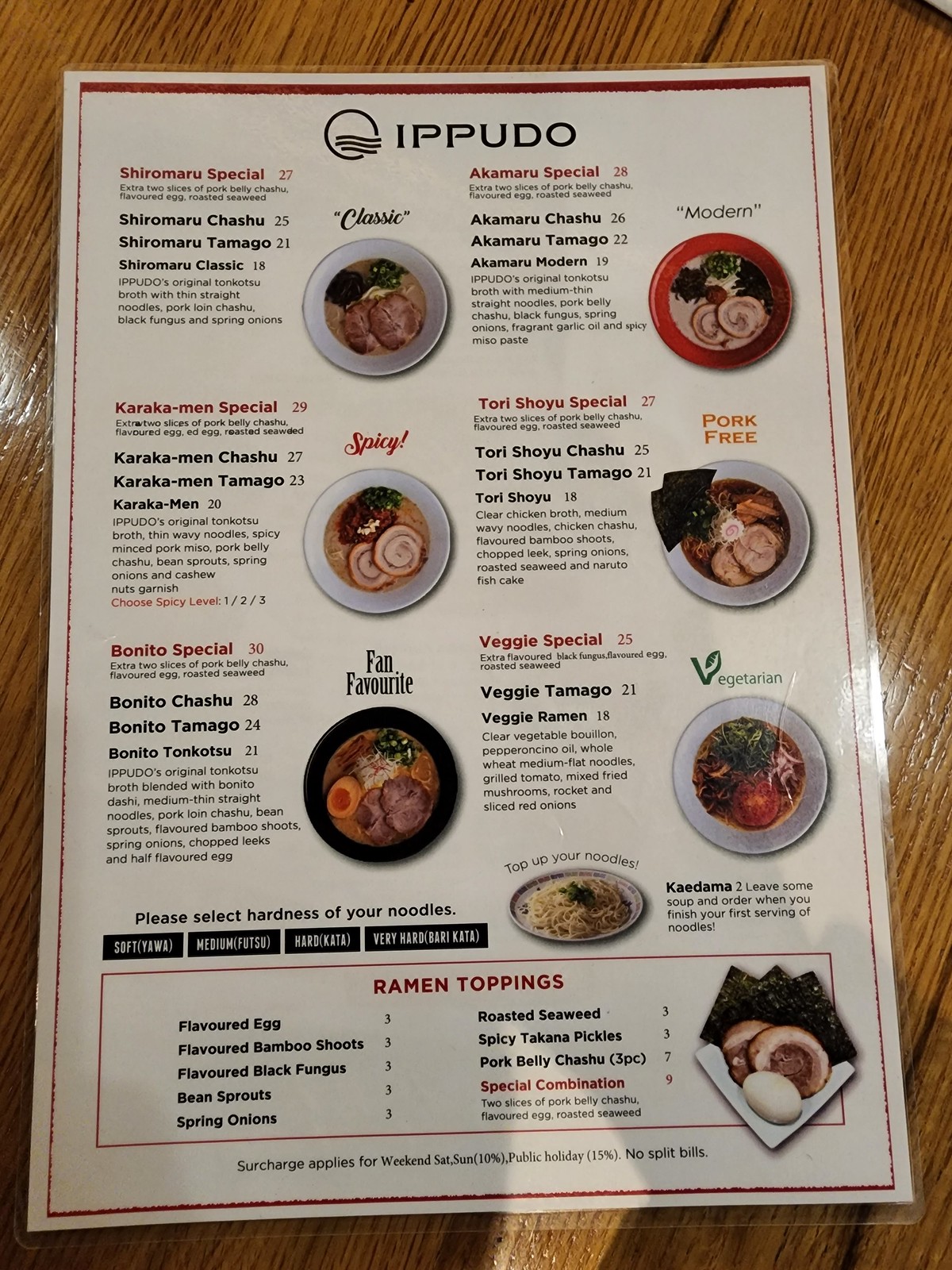A close-up photograph showcases a well-laminated menu from the renowned ramen restaurant, Ippudo, displayed on a rustic wooden table surface. The menu prominently features vibrant images of various ramen dishes available for order, including the Shiro Maru Special, Akemaru Special, Karakamen Special, Tori Shoyu Special, Veggie Special, and Bonito Special. Each dish is visually detailed, suggesting an array of ramen options catering to different tastes. Customers are also invited to personalize their ramen with a selection of additional toppings. The photograph appears to have been taken from a top-down perspective, capturing a faint shadow from the person standing above, adding a subtle depth to the image. The overall arrangement beautifully contrasts the rich, appetizing details of the menu against the natural wood grain of the table.